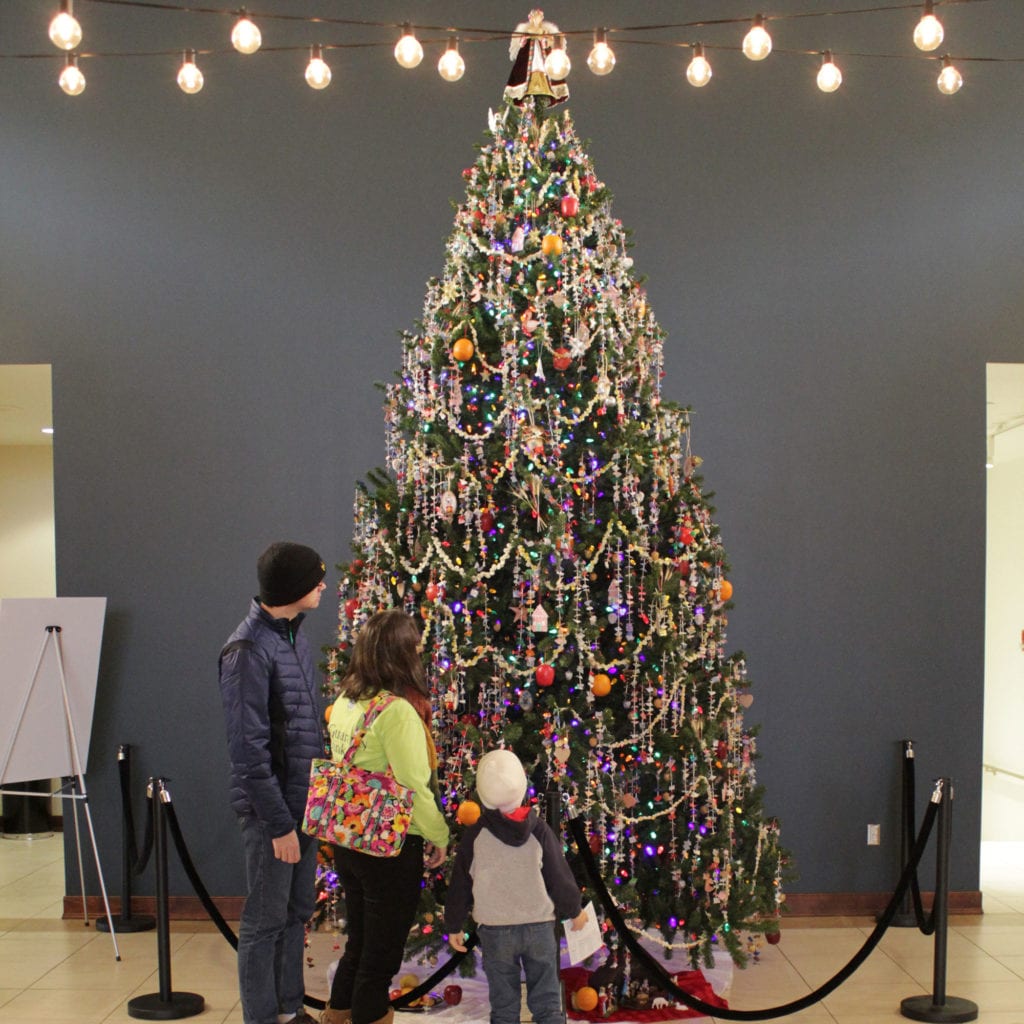This image captures a magnificent, heavily decorated 12-foot Christmas tree standing tall indoors, possibly in a church, mall, or museum. The tree reaches almost to the ceiling and is adorned with an abundance of ornaments, glittering lights, streamers, and garlands, including strings made of popcorn and beads. Uniquely, there appear to be fruit ornaments like oranges hanging from its branches. The space behind the tree features a plain dark blue wall and is lit by round string lights hanging from the ceiling.

In the foreground, a family of three stands in awe, gazing up at the tree. They are dressed in winter clothes: the father on the left is in a black beanie, navy puffy jacket, and blue jeans; the mother in the middle dons a light green long-sleeve shirt, black pants, and carries a colorful bag on her right shoulder; while their young daughter stands between them. The entire scene is roped off with a black cord, hinting that this stunning tree is part of an exhibit. A white sign near the entrance of the roped-off area, though not facing the viewer, possibly provides details about the display.